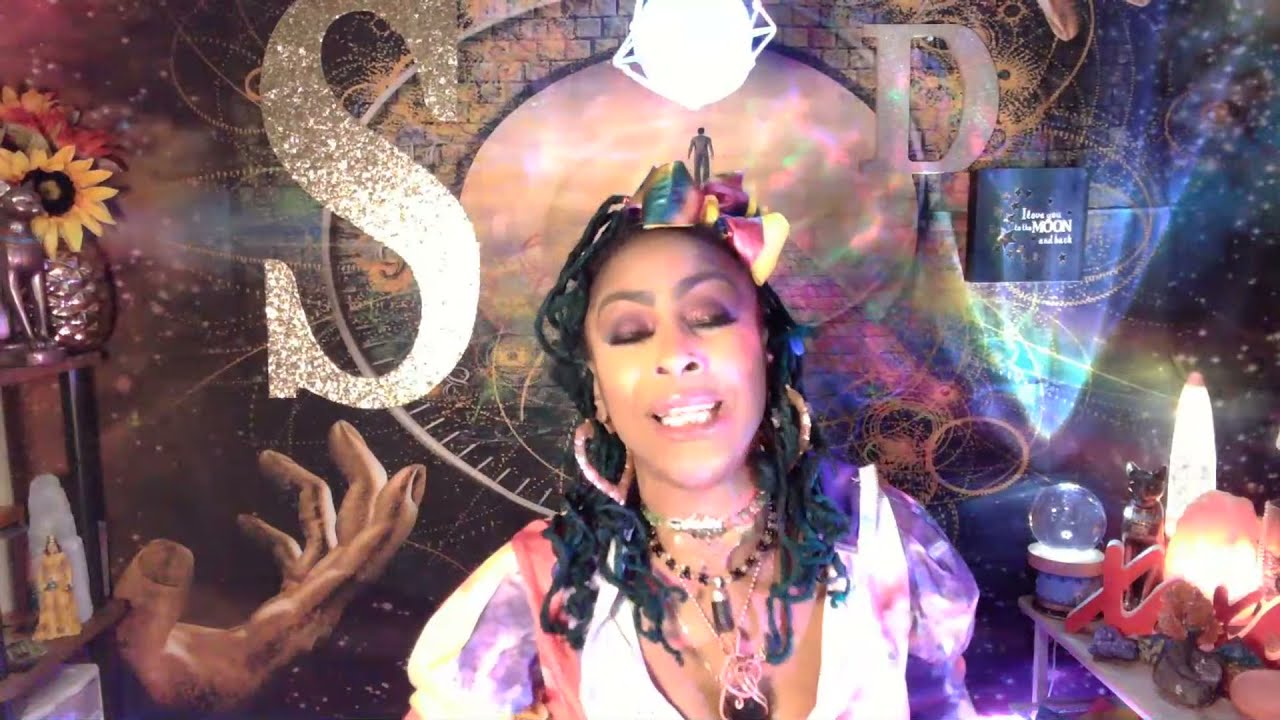The image is a detailed, photoshopped collage of an African-American woman depicted from the chest up. She has curly black hair adorned with a large, rainbow-colored bow featuring swirly patterns of pink, yellow, green, and blue. Her oversized pink heart-shaped hoop earrings dangle prominently against her shoulders. The woman is attired in a vibrant tie-dye blouse with shades of purple, white, and pink, possibly accessorized with pink suspenders. She is adorned with an impressive array of necklaces—five to seven in total—some of which are short and tight around her neck, while others drape elegantly into her cleavage, featuring stones or perhaps small potion bottles.

Her face is expressive, captured with her eyes closed, showcasing her mascara, eyeliner, and neatly adjusted eyebrows. Her mouth is slightly open, giving the impression that she might be speaking or singing.

The backdrop adds to the mystical aura of the image, featuring an eclectic mix of New Age symbols and letters, including a large glittery gold "S" and a "D." The colorful mural behind her includes a black starry sky, an outreached black hand, various crystals, flowers, and a globe. There is also a small wooden shelf in the lower right corner, holding a snow globe and a glowing salt rock lamp, emphasizing the mystical, fortune-teller-like setting that also includes elements of glowing lights and potentially even a lava lamp.